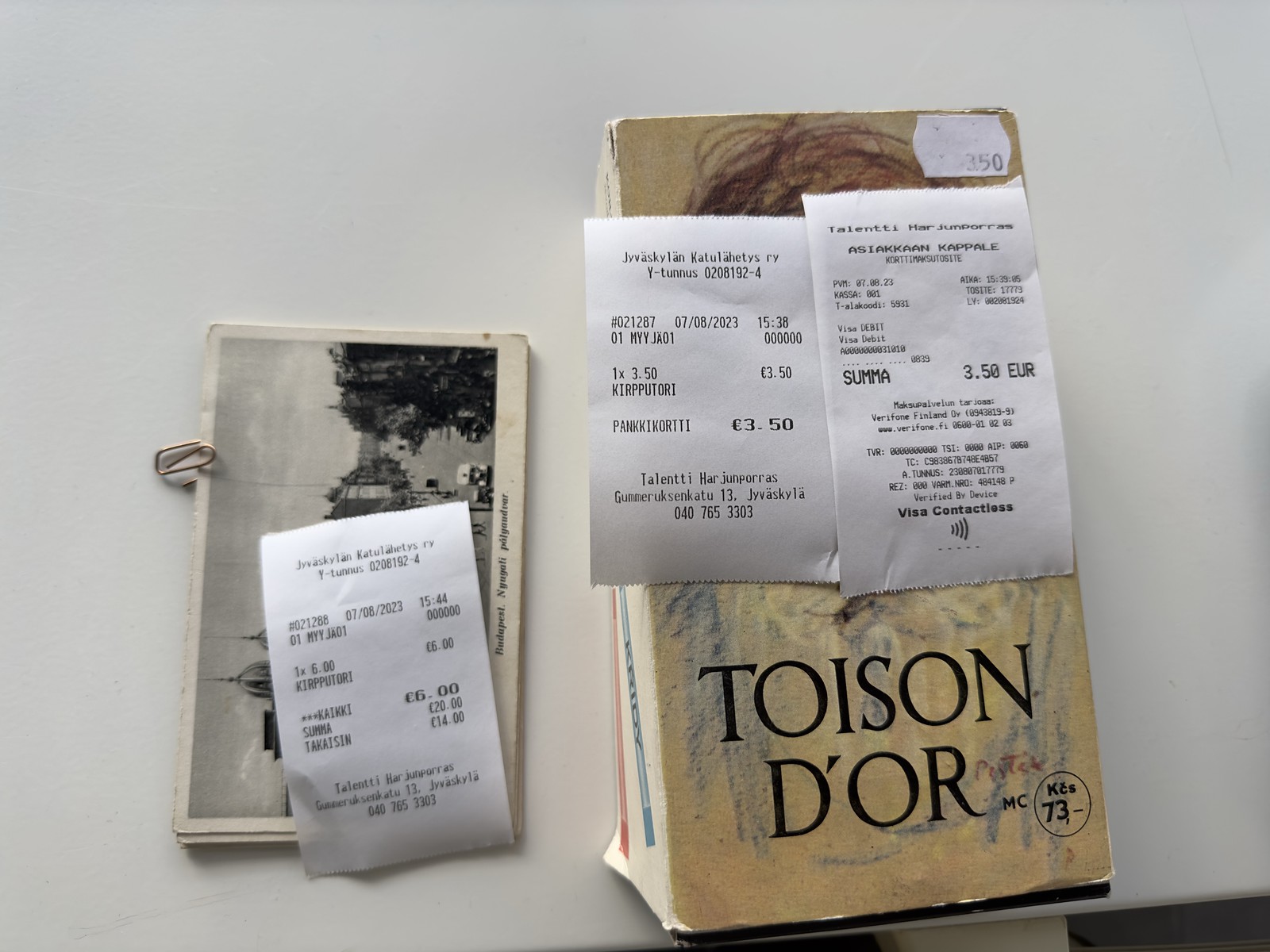This color photograph features an intricate tableau of old black-and-white postcards and a stack of books, all entwined with several white till receipts. On the left, the postcards are clipped together by a silver paper clip, partially obscured by a receipt dated August 7, 2023, at 15:44, detailing amounts such as £1 times $6, £6, £20, and £14. To the right, the stack of books includes a top book covered by two overlapping receipts. The book's cover, primarily cream-colored, bears the black text "TOISON D'OR" with a circular logo featuring "MC" and "KCS 73." The receipts exhibit various details in a foreign language, including the word "SUMMA" suggesting a summary, with totals such as 3.50 EUR and Visa contactless payment symbols. Adjacent to this, a brown cardboard box is whimsically adorned with crayon drawings in light blue and black, partially hidden under more receipts. A sticker marked "350" and additional black lettering embellish the box, adding to the rich tapestry of this seemingly mundane yet captivating still life.